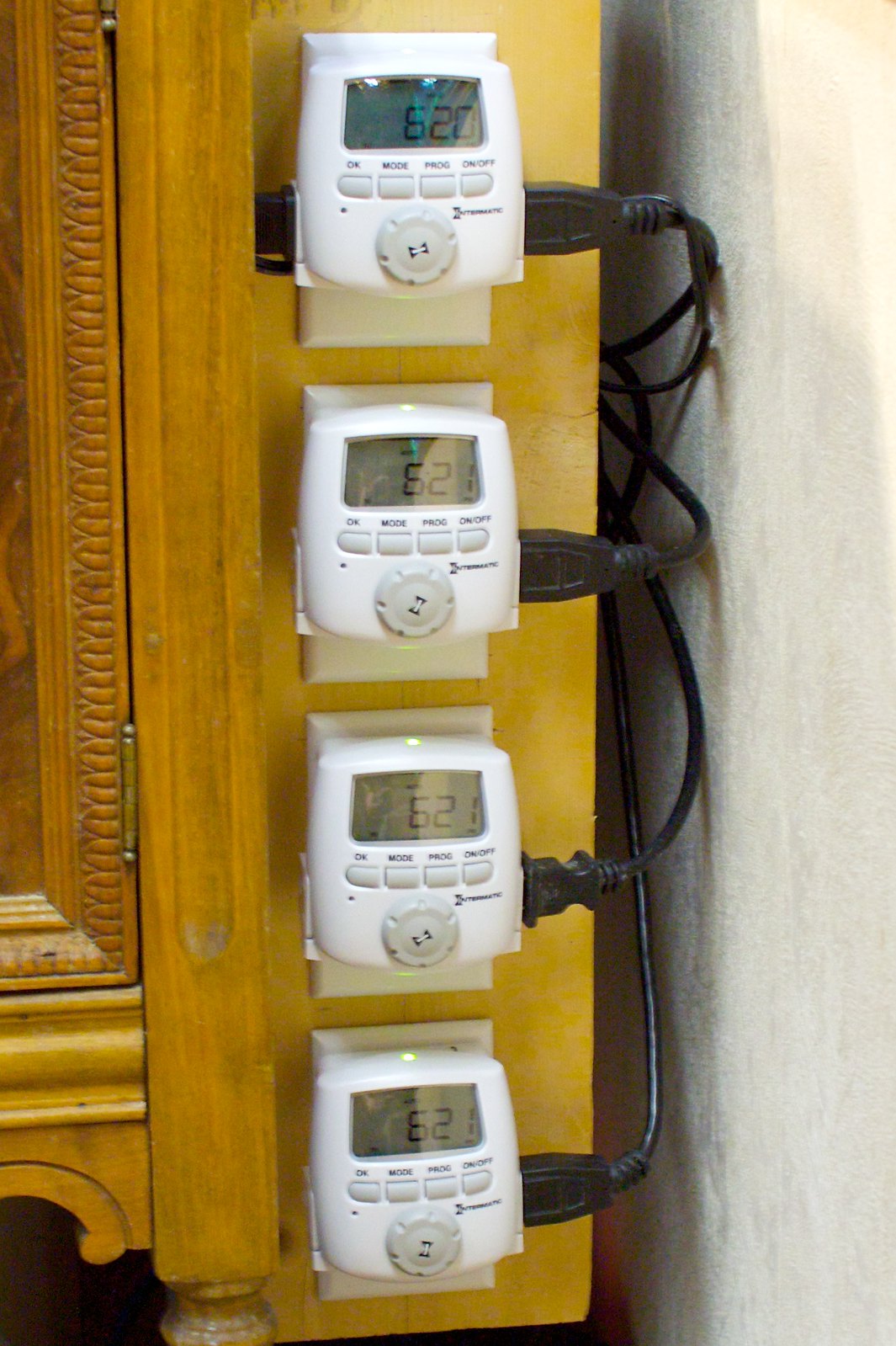In this image, we observe four digital timers positioned against a piece of furniture, likely a desk or table made of yellowish-brown wood. Each timer features an LED display, with the top one reading "6:20" and the three below it showing "6:21." The top timer has two black plugs inserted—one on the left side and one on the right—while the lower three timers each have a single plug on the right side. The connecting wires trail along the right side, disappearing behind the furniture.

The furniture appears to be up against a white wall, with bronze-colored hinges visible on its door. The door features decorative grooves and is cut off at the bottom of the image. The base of the furniture has rounded edges, creating a small clearance underneath.

Each timer is equipped with four white buttons aligned horizontally beneath the LED displays, accompanied by labeled text above them. Below these buttons is a central dial. A red light is visible in the bottom right corner of the image, adding a subtle glow beneath the timers. These timers seem to be plugged into a panel occupying four wall outlets.